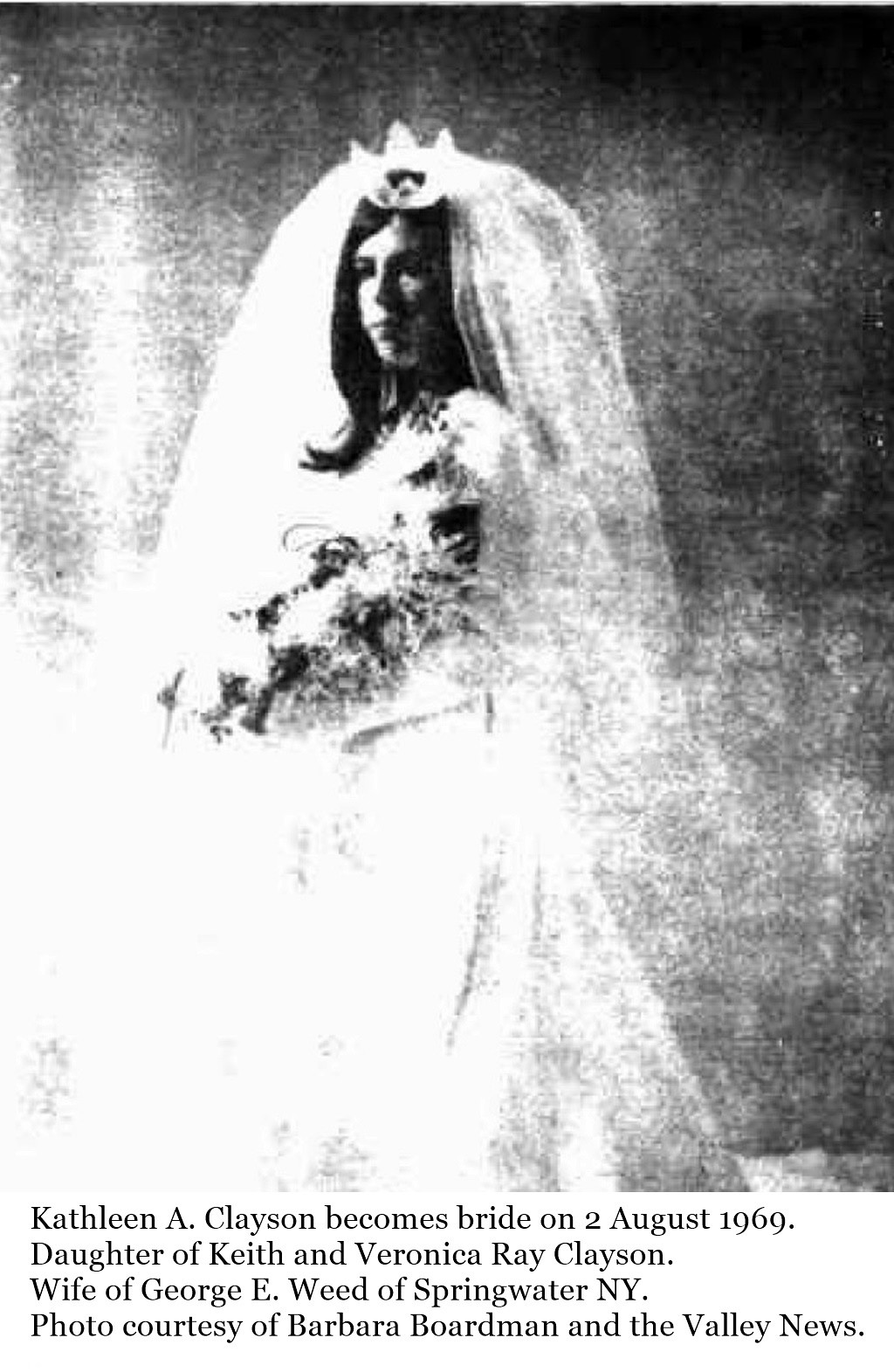The image is a black-and-white photograph that appears to be an old newspaper clipping, notable for its blurry and low-quality scan. The main subject of the photo is a bride named Kathleen A. Clayson, who became a bride on August 2nd, 1969. The text below the photograph identifies her as the daughter of Keith and Veronica Ray Clayson and the wife of George E. Weed from Springwater, New York. The photo is credited to Barbara Boardman and the Valley News.

Kathleen is dressed in a traditional white bridal gown that has an extremely long train, reminiscent of Victorian-era styles. She holds a large bouquet of flowers, with some flowers appearing red despite the black-and-white format. She has long, dark hair that cascades past her shoulders and wears a white headdress that looks like a crown at the top of her veil. The lighting in the photograph creates a high contrast, making the bottom left of the image very bright and white, while the top right is notably darker, adding a ghostly effect to the picture. Overall, the image captures a momentous occasion in a somewhat ethereal and nostalgic manner.